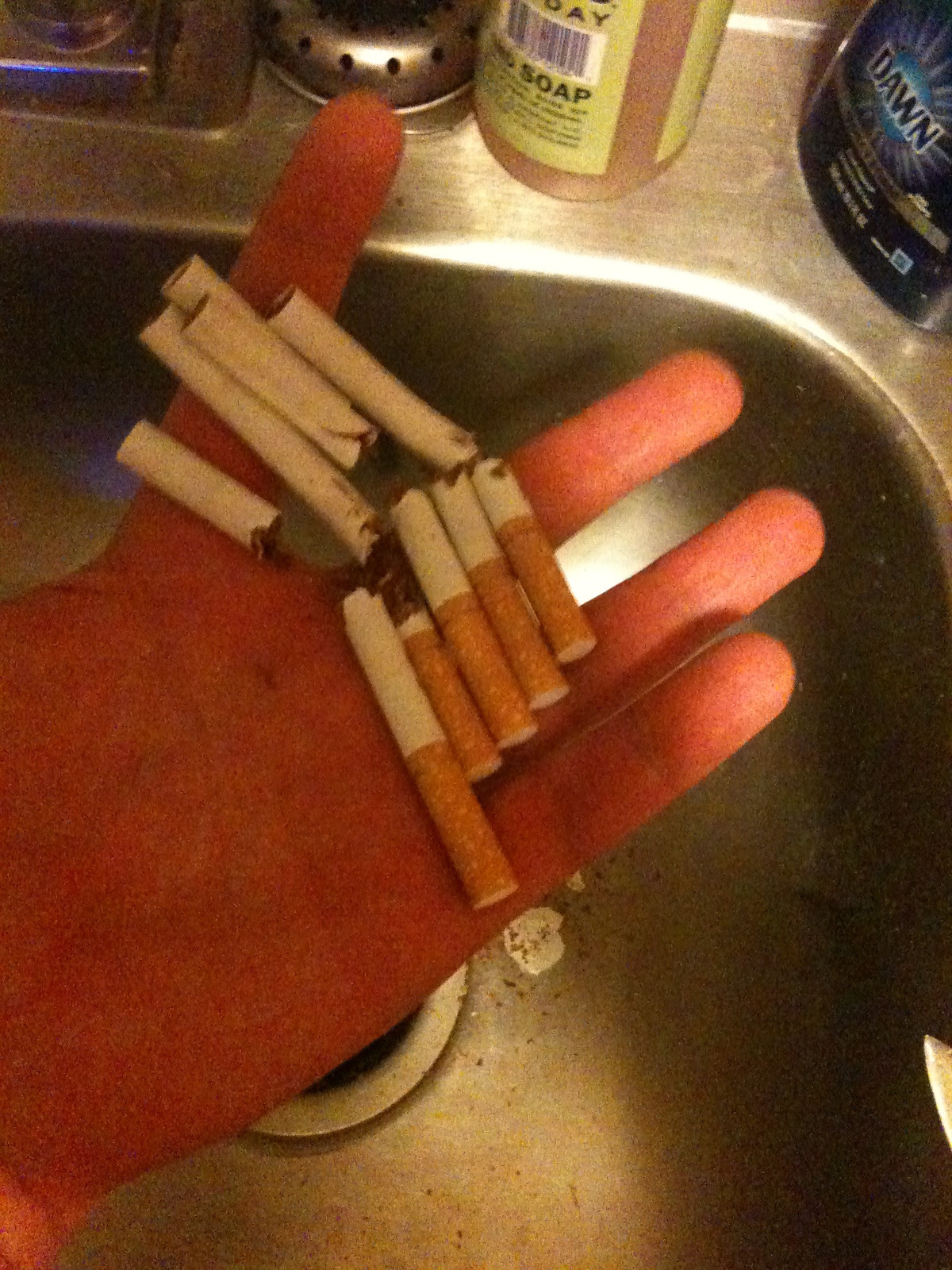This close-up photograph captures the left hand of a person, possibly of European descent, holding five broken cigarettes over a stainless steel kitchen sink. The cigarettes are filtered, with light brown filters and white casings, all broken in the middle, resulting in tobacco debris scattered in the lower part of the sink. The hand, positioned under yellow lighting, appears very red, with four visible fingers and the thumb obscured. In the upper right corner of the image, a blue bottle of Dawn dishwashing detergent and a tan-colored hand soap are positioned next to each other, with a sink stopper noted to the left of the soap containers. The photo is taken from an upper view, emphasizing the scene's various elements and the fragmented cigarettes against the metallic basin.